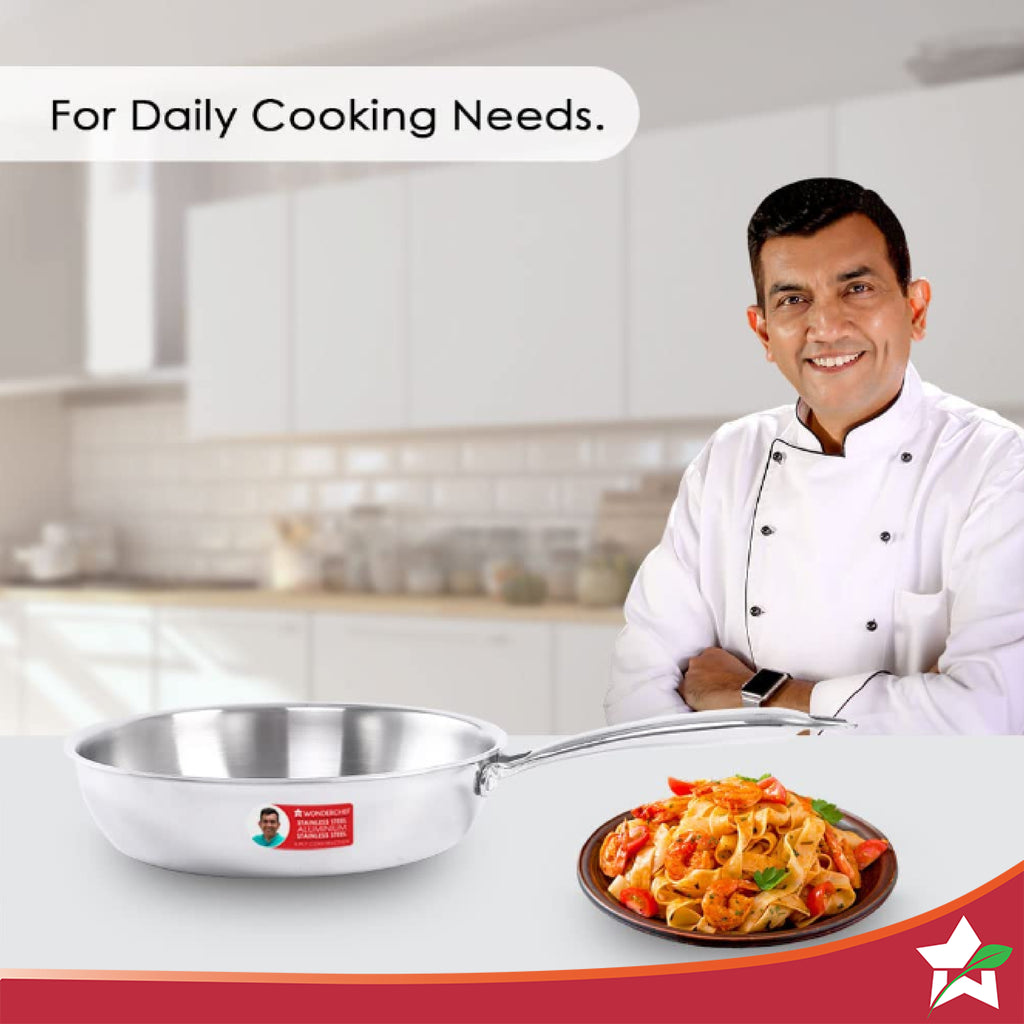The advertisement features a vibrant kitchen backdrop that is slightly blurred to highlight the central elements. Prominently positioned on the right side is a smiling Latino chef, dressed in pristine white chef's attire with classic buttons, a neatly greased-back, black hairdo, and a watch on his wrist. The chef's friendly demeanor sets a welcoming tone for the ad. 

Positioned on the left side of the image is a sleek, silver skillet with the chef's face imprinted on a sticker. Adjacent to the skillet, and taking up the lower right portion of the ad, is a delectable plate of pasta, adorned with seafood, red peppers, and cheese, presenting a colorful array of yellow, red, and green hues. 

The top left corner of the ad showcases the slogan "for daily cooking needs" in bold black lettering against a clean white background. At the bottom, a burgundy banner with orange edging spans across, culminating in the company's logo in the lower right corner - a white star with a green leaf draped across it. The blended elements of the chef, kitchen, and cookware create a cohesive and enticing visual that emphasizes the quality and reliability of the advertised culinary products.